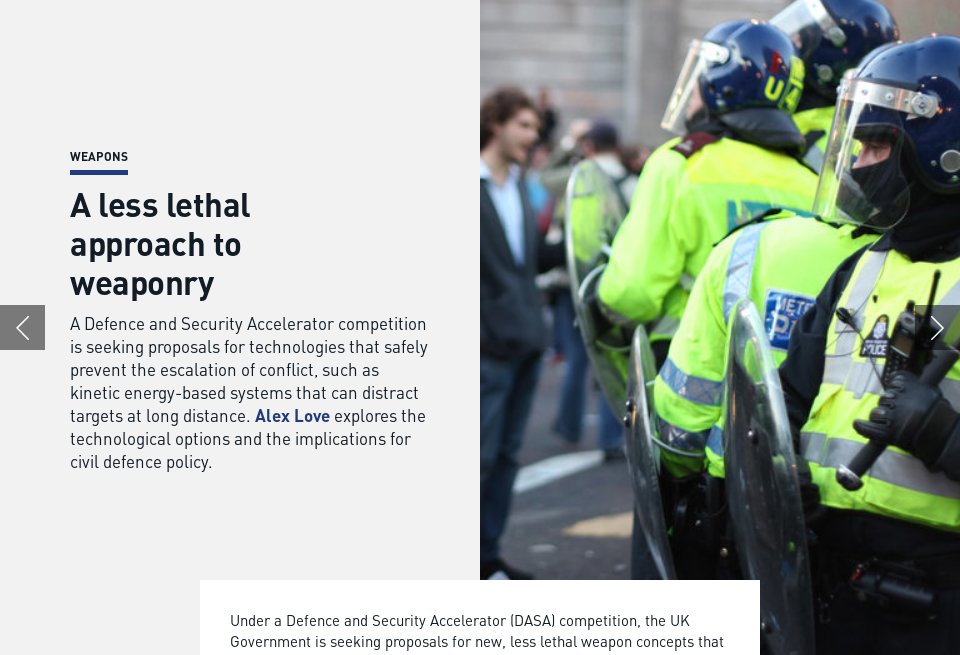The image is a screenshot of a section of a website focusing on defense and security innovation. On the right side, there is a picture depicting law enforcement or security personnel equipped with riot shields and helmets, indicative of a crowd-control scenario. To the left, slightly above the middle of the image, there's a bold heading that reads "Weapons". Directly beneath, the title states "A Less Lethal Approach to Weaponry". The accompanying text outlines a defense and security accelerator competition seeking proposals for technologies aimed at preventing conflict escalation through non-lethal means. It highlights kinetic energy-based systems designed to distract targets from a distance. The text continues with "Alex Love" in blue, followed by "explores the technological options and the implications for civil defense policy" in black. Below the main text, there's a condensed version of the paragraph, suggesting a summary or introduction to the article's content. The overall layout and terminology suggest that the context is UK-based.